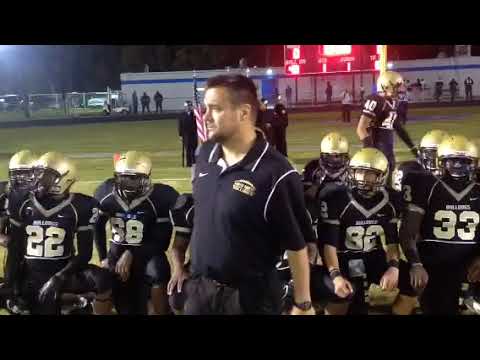This horizontally aligned rectangular photograph, framed by thick black borders at the top and bottom, depicts a somewhat blurred scene involving a high school football team. The players, identifiable by their gold helmets and dark-colored uniforms with gold trim, are kneeling on one knee on a light green field marked with white stripes, suggesting their position in the end zone. Prominent among the players are those with visible numbers: the young man in the middle sporting number 5, flanked by number 16, and another wearing 85 or 65. Their coach, dressed in a matching dark short-sleeved top, stands with his back to the camera, addressing the team with a rolled-up play call sheet sticking out of his back pocket. In the background, an inflatable mascot head resembling a bulldog, with big teeth and a brown side, hints at the team's possible nickname, the Bulldogs, and their spirited entrance tradition.